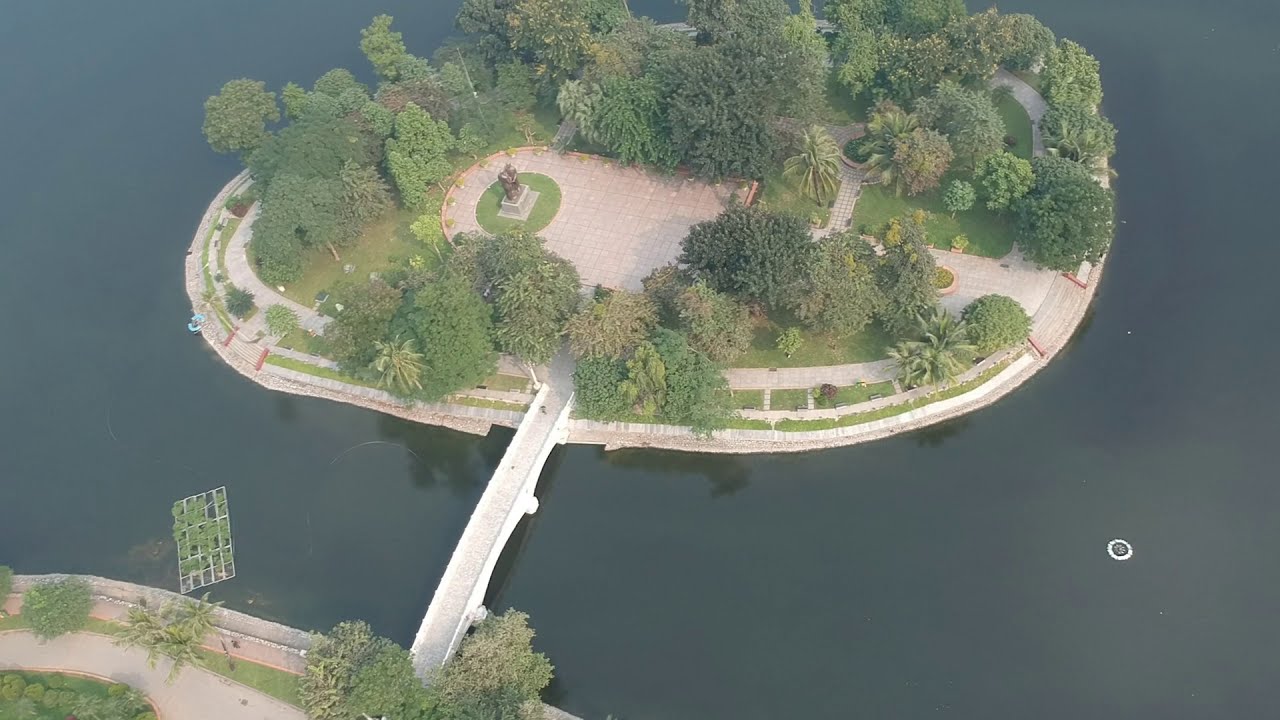From an aerial perspective, we see a serene island in the middle of a calm, greenish body of water. The island boasts an oval shape, with its edges sharply defined where the water meets the land. Central to the island is an open space adorned with orange-colored tiles that form a shape flat on the right side and curved on the left. At the heart of this tiled area stands a bronze-colored statue atop a gray pedestal, encircled by a green lawn. Surrounding the central area, tall and dense green trees dominate the landscape, though there are a few patches of visible green grass. A light brown bridge with white barriers extends from the island, connecting it to a nearby landmass. On the bottom left of the image, this piece of land features a light gray walkway accompanied by green vegetation and a couple of green bushes. Another feature in the water on this side is a rectangular shape with white bars and green vegetation growing through it. The overall scene suggests a tranquil and scenic area, ideal for leisurely walks and appreciation of natural beauty.